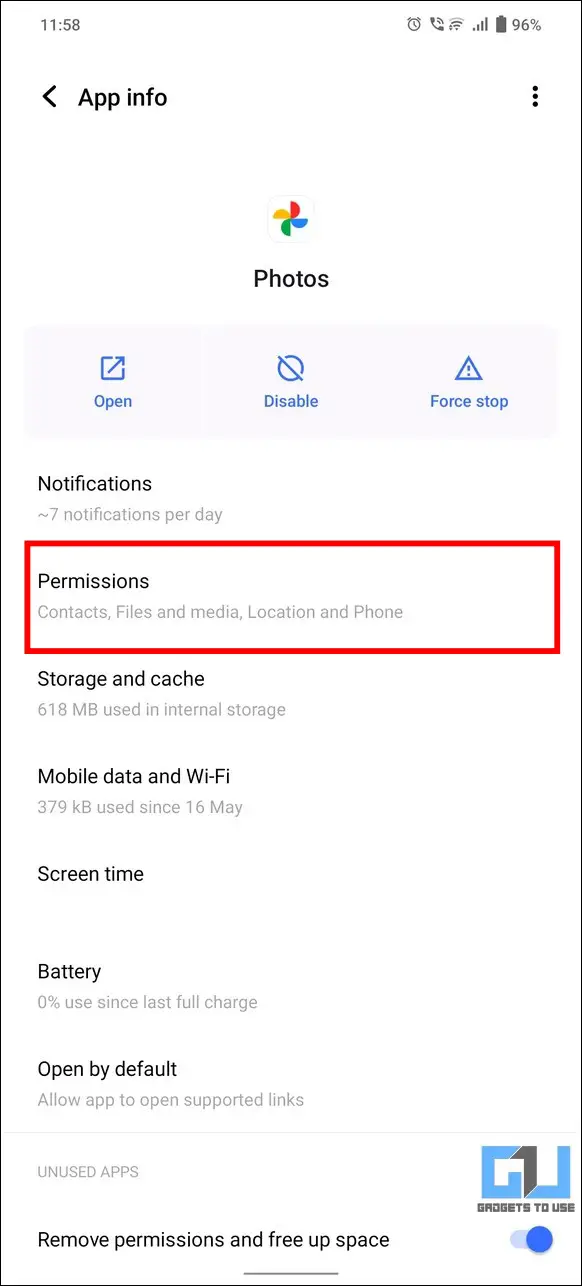The image shows a screenshot of an app information sub-menu on a smartphone with a white background. At the top of the image, the device's status bar displays the time as 11:58 beside icons for a clock, phone, and a battery with a 96% charge. Below the status bar, in black text, is the label "App info" accompanied by a back button on the left and three vertical dots on the right, indicating more options.

Centered on the screen is the app's name "Photos" accompanied by a multicolored whirly icon in shades of red, gold, green, and blue. Below the app icon, there are three blue buttons: "Open" (represented by a square with an arrow), "Disable" (symbolized by a circle with a slash through it), and "Force stop" (marked with an exclamation mark).

The main section of the screen is black, detailing various app settings:
- **Notifications**: Displays "7 notifications per day".
- **Permissions**: Highlighted with a red box, it lists permissions for Contacts, Files and Media, Location, and Phone.
- **Storage & cache**: Indicates "618 MB used in internal storage".
- **Mobile data & Wi-Fi**: Shows "379 KB used since 16th May".
- **Screen time**: Not elaborated.
- **Battery**: States "0% used since last full charge".
- **Open by default**: Allows the app to open supported links.
- **Unused apps**: Includes options to "Remove permissions and free up space".

A gray divider line separates the above details from additional elements at the bottom. To the left side at the bottom, there are blue and gray letters, possibly "G" and "U," with small gray text beneath them. Below this text, a blue circle is visible.